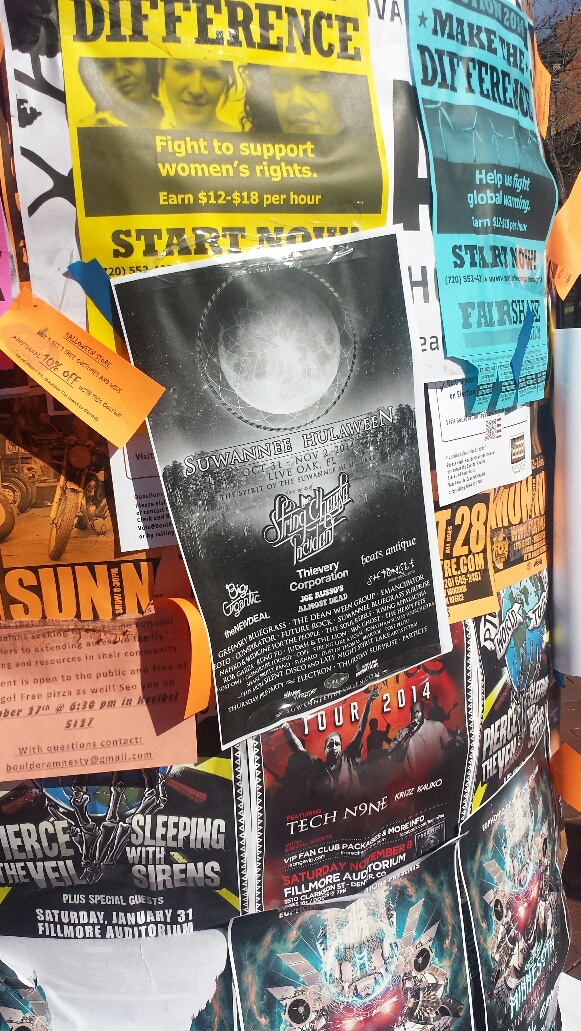The image depicts an outdoor community bulletin board or possibly a light pole plastered with a dense collection of overlapping and layered advertisements and posters in various colors and styles. Prominent among these is a yellow flyer in the center with black text that reads, "Difference. Fight to support women's rights. Earns $12 to $18 an hour. Start now." There is also a light blue handbill nearby with the phrase, “Make the Difference. Start Here.” 

Surrounding these key posters are a multitude of other ads, some of which are partially obscured. These include an orange announcement, a vibrant tour poster from 2014 featuring Tech N9ne with ghoulish figures, and several concert promotions including names like "Sleeping with Sirens." The display is a vivid patchwork of blue, yellow, red, green, and orange hues, creating a visually noisy and colorful collage of calls to action, events, and causes. The posters seem to have accumulated over time, forming a chaotic yet vibrant mosaic of community messages and advertisements.